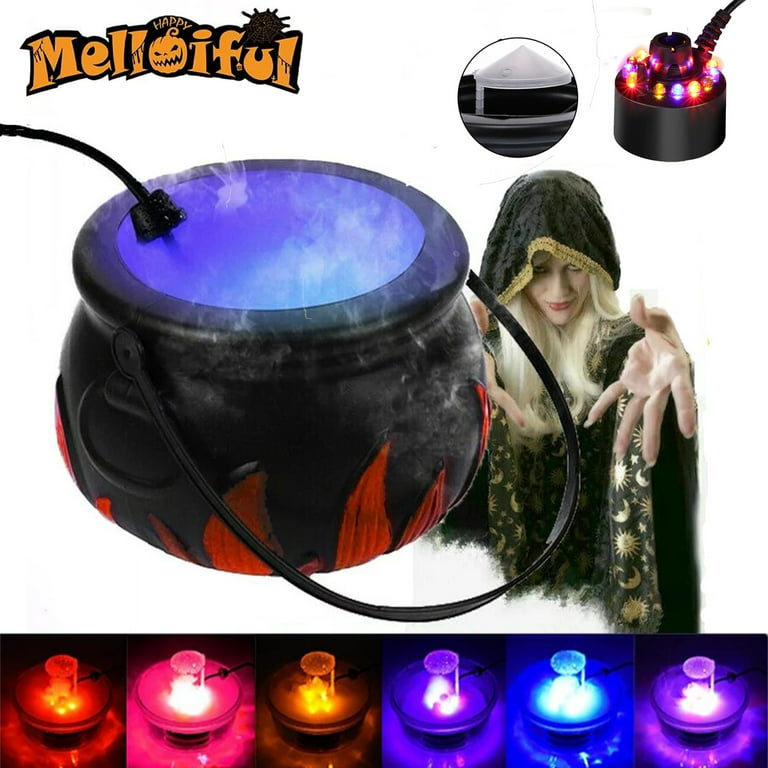The image showcases a Halloween-themed product called "Meloiful," prominently displayed in vibrant orange text with a jack-o-lantern design substituting the "O." The centerpiece of the image is a detailed color photo featuring a small, black plastic cauldron with painted red flames and a handle. The cauldron emits a fog from a connected tube and is illuminated by interior LED lights in various hues. Behind the cauldron, a woman dressed as a witch, in a cloak adorned with stars and moons, stands with her hands outstretched, beckoning the viewer. In the top right, zoomed-in circles highlight parts of the device, including a cylindrical component with an electrical plug and colored LED lights. Below, the image displays six smaller photos arranged in a row, showing the different color variations the cauldron can change to: red, pink, orange, blue, darker blue, and purple.